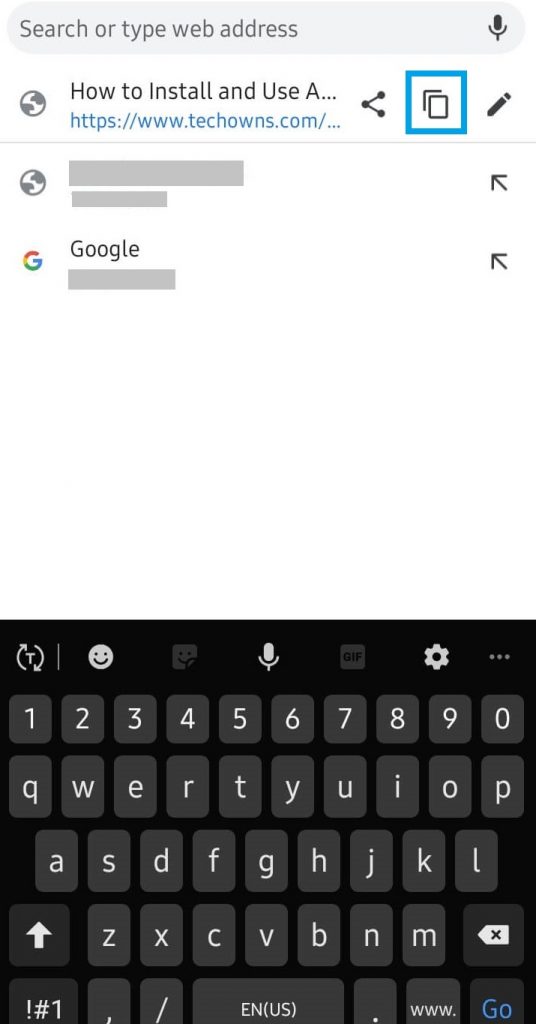A detailed and polished caption for the image might look like this:

---

A screenshot of a mobile phone display captures a user actively engaged in a web search. The device's keyboard is visible at the bottom of the screen, ready for input. The search interface is minimalist, lacking the usual task bar details such as time, battery life, or signal strength indicators. At the top, a gray search bar with darker gray text prompts, "search or type web address," accompanied by a microphone icon on the far right.

Below the search bar, various search suggestions and results are listed. The first result is partially visible, displaying the beginning of the query "how to install and use" from https://www.techowns.com. This entry is marked with an RSS feed-like icon, an overlapping squares icon, and a blue outlined rectangle with a pencil icon beside it.

Further down, there is another search result, but its text is censored and unreadable. This is followed by a censored Google search result. Both of these censored entries have small arrows pointing diagonally to the top left, located on the far right side of the entries. The rest of the screen does not feature any additional elements.

---

This caption provides a detailed description of the image while maintaining clarity and structure.